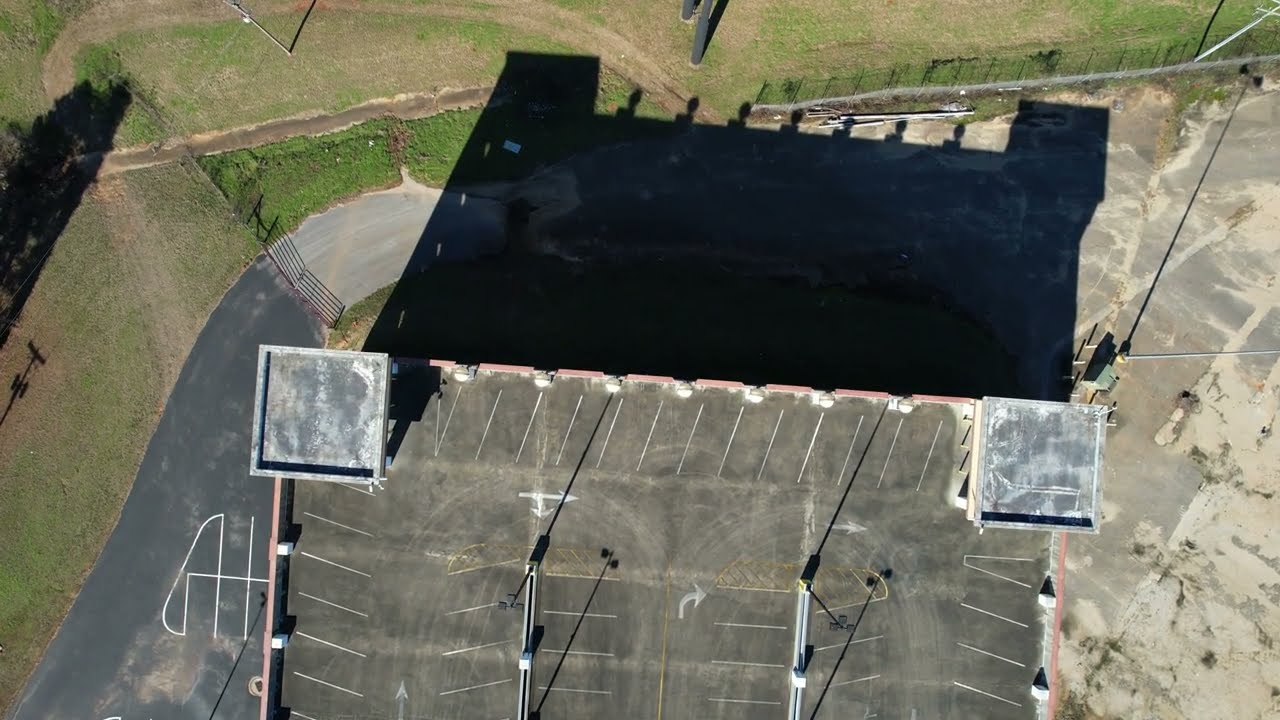An aerial photograph captures an overhead view of a parking structure, suggesting it may be linked to a prison complex. The parking structure is square in shape with two additional square watch towers positioned on its left and right corners, casting long, ominous shadows toward the upper part of the image. The structure's light beige and gray asphalt surface is marked with white parking lines and shows signs of wear with old and broken pavements. Adjacent to the parking structure, on the left side, is a narrow paved road, while on the right is a dilapidated parking lot, characterized by multiple worn-out pavements and visible foliage sprouting through cracks. Surrounding the parking structure, particularly on the upper and left sides, is a sprawling field of grass varying in shades of dark and light green interspersed with patches of brown. A brown path meanders through this field. Encircling the entire area is a fence, backed by the larger main building with spotlights, reinforcing a sense of surveillance and security. The entire scene underscores a tightly controlled environment likely designed to prevent escapes.